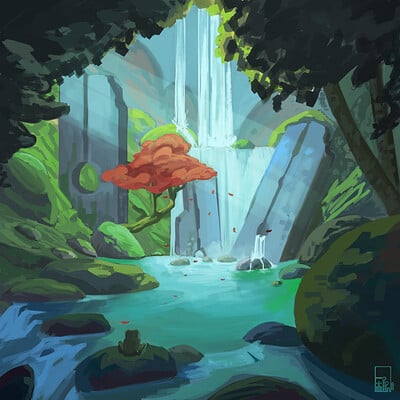The image is a detailed digital illustration portraying a series of cascading waterfalls within a lush, forested landscape. The composition is square, with a massive body of light blue water in the center, transitioning to greenish hues near the edges. In the foreground, scattered stones lead to a smaller waterfall on the lower left, while two circular green boulders rest on the right side. Prominent brown tree trunks rise from the boulders, crowned by a dense mass of green leaves. 

On the left, a hilly terrain with darker leaves and a noticeable tree with red foliage adds depth to the scenery. This tree stands near an apparent door embedded in the cliff. The background features a multi-level waterfall system; the initial waterfall flows into a second, larger one beneath it, with white water cascading down from an unseen source above. The scene is enveloped in shades and shadows, with cliffs and rocks enhancing the rugged beauty. Rounding out the natural ambiance, soft rays of sunlight pierce through the upper left, illuminating the scene and casting a serene glow.